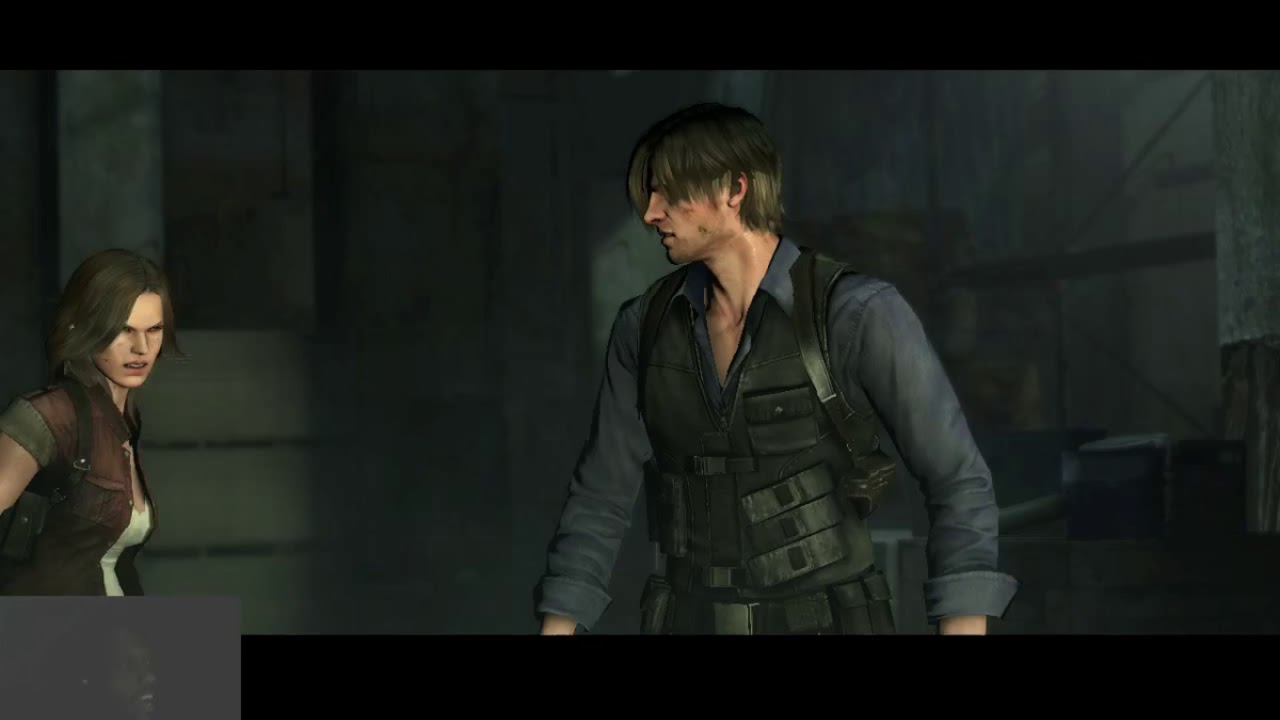This image appears to be a dark, atmospheric scene from the video game Resident Evil 6, featuring the characters Leon Kennedy and his partner. The setting is an indoor, dimly lit area, with a letterboxed format showing black bars at the top and bottom of the screen, as well as a gray box in the lower left corner that appears to display a streaming overlay featuring a black man's face.

In the center of the image stands Leon Kennedy, identifiable by his long blue collared shirt with the cuffs rolled slightly up his wrists. He wears a black tactical vest with multiple pockets and compartments, and a leather gun holster slung over his left shoulder, possibly also his right. Leon's hair is shaggy with a 90s mushroom cut appearance, and his face shows signs of being dirty and scratched, indicating recent combat or a tough journey. His sweaty, glistening skin suggests he's either gearing up for a confrontation or recovering from one.

To Leon's left, on the viewer's right side, is his partner, who is seen wearing a red vest jacket over a white top. Her hair is long, and she seems less beaten-up compared to Leon but clearly shares in the stressful circumstances. She also has a weapon holstered around her shoulder, highlighting the dangerous environment they are navigating. The background features the gray walls of an interior building, enhancing the ominous and tense aura of the scene.